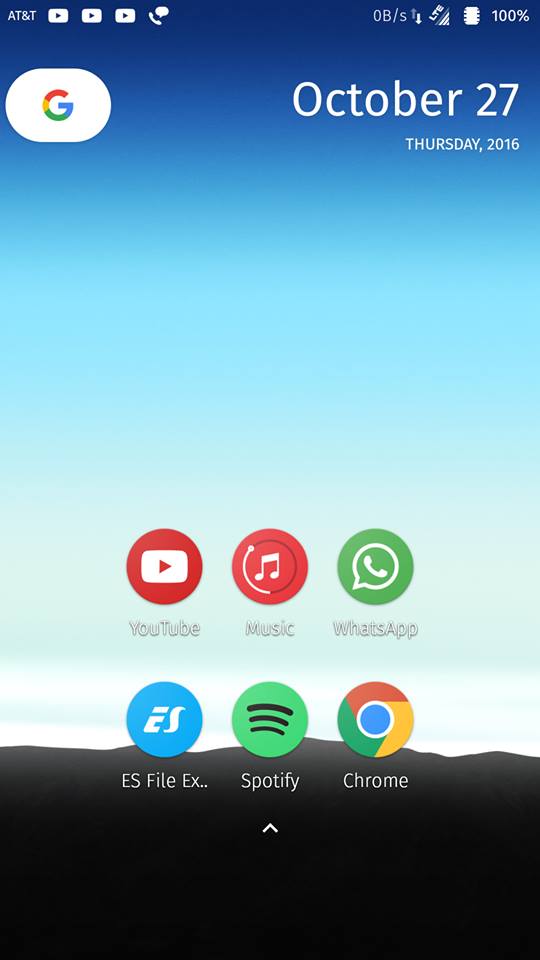This image depicts the home screen of an Android device, identified by the prominent Google icon in the top left corner. The background wallpaper showcases a scenic sky, transitioning from a dark charcoal hue at the very bottom, which suggests ground or mountains, into white clouds. As your eyes ascend, the sky shifts from a light blue to an aqua blue, culminating in a deeper blue at the top.

At the top of the screen, there is an AT&T logo to the left, indicating the network provider. Right next to the logo are three YouTube notification icons and a WhatsApp notification icon, followed by the text "OB-S." Additionally, there are two arrows, one pointing upwards in gray and another downwards in white, next to the text "LTE," arranged in a diagonal fashion with the "L" angled towards the bottom left. Signal strength bars indicate three out of four bars, and a battery icon shows a full charge at 100%.

Centered on the screen, there is a widget displaying the date. It features a rounded rectangle with a sharp white background and white text that reads "October 27th" in bold letters and "Thursday, 2016" in a smaller, thinner font.

The lower section of the screen is populated with various app icons. In the bottom left corner, there is the YouTube app icon with "YouTube" written below it in white text, accompanied by a subtle gray or black shadow. To the right is the music app icon, depicting a musical note within a circular progress bar surrounding it. Next to it is the WhatsApp app icon.

On the following row, the ES File Explorer app is represented by an "ES" logo within a blue circle, captioned "ES File X.." Further to the right are the Spotify app icon and the Chrome browser icon.

Situated at the very bottom of the screen is an upward-pointing arrowhead in white, signifying additional options or a hidden app drawer.